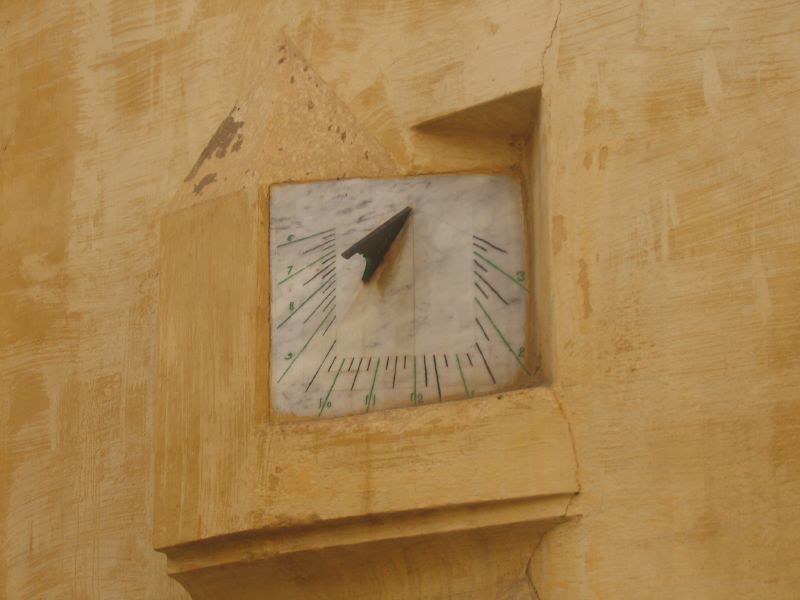In this intriguing image, we see an unusual clock seamlessly integrated into a panel made of light-colored wood, allowing the natural wood grain to subtly enhance its surface. Embedded within the wooden structure, which might be part of a larger wooden bookcase or chest, lies an ivory-colored tile serving as the clock face. This clock face deviates from traditional design, presenting its numbers in a unique formation: they commence from one side, continue along the bottom, and rise up the opposite side, leaving the top area devoid of any numerals. A single black arrow serves as the clock's hand, indicating the current time in this unconventional, yet fascinating setup. The overall aesthetic harmoniously blends the organic texture of the wood with the distinctive clock design, making it a compelling focal point.